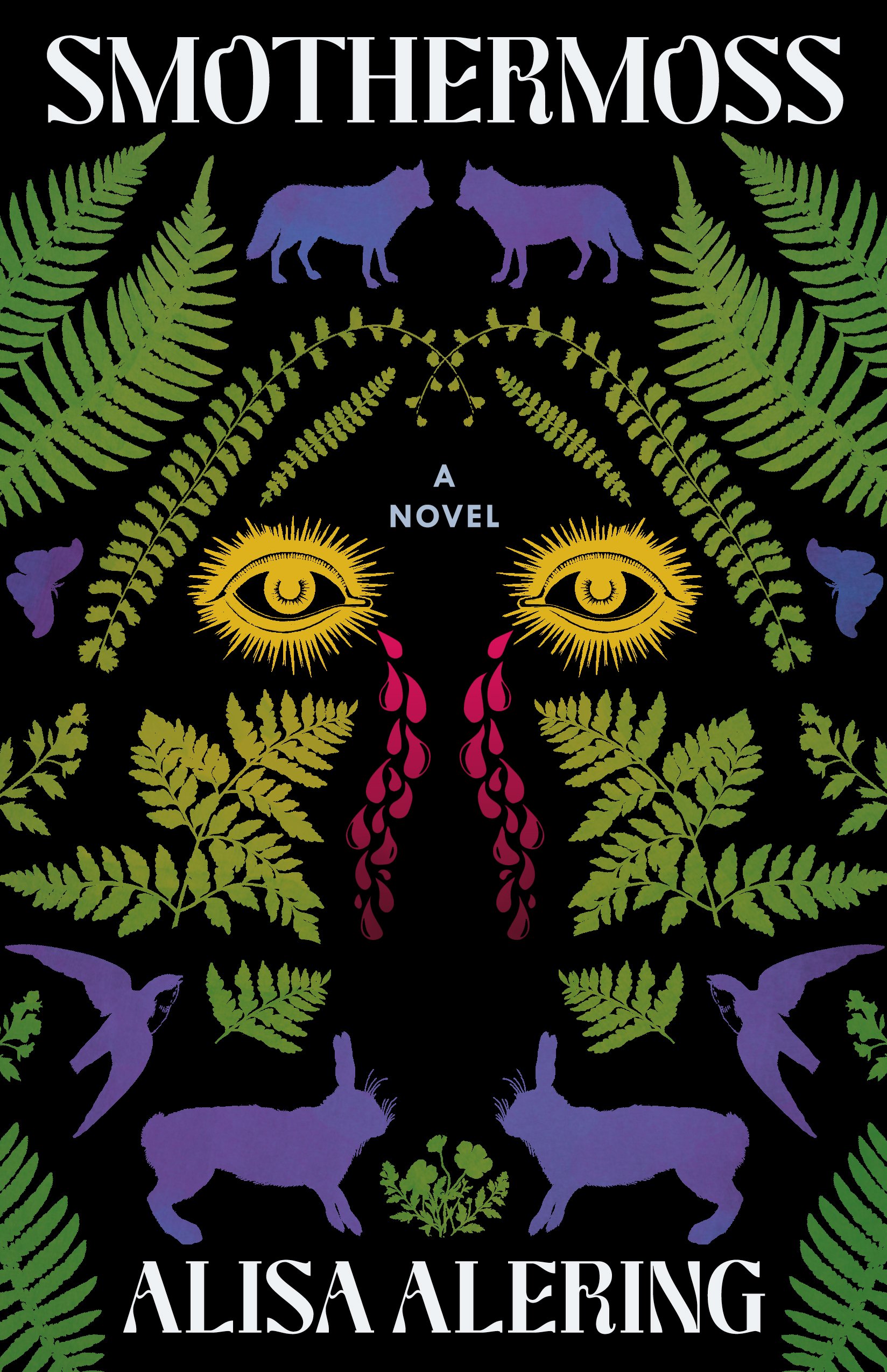The image is a highly detailed and captivating book cover for the novel "Smother Moss" by Alyssa Alluring. Set against a black background, the title and author's name are prominently displayed in white lettering, with "A Novel" in smaller text. The cover features an intricate collage of plants and animals that form the outline of a mysterious figure. Among the greenery, which includes vibrant green ferns, are various animals depicted in purple, such as wolves, rabbits, birds, and a dog, along with distinct yellow eyes and a red nose that stand out in the center. The eye-catching design, with its mix of vivid colors and detailed natural elements, invites curiosity about the story within.